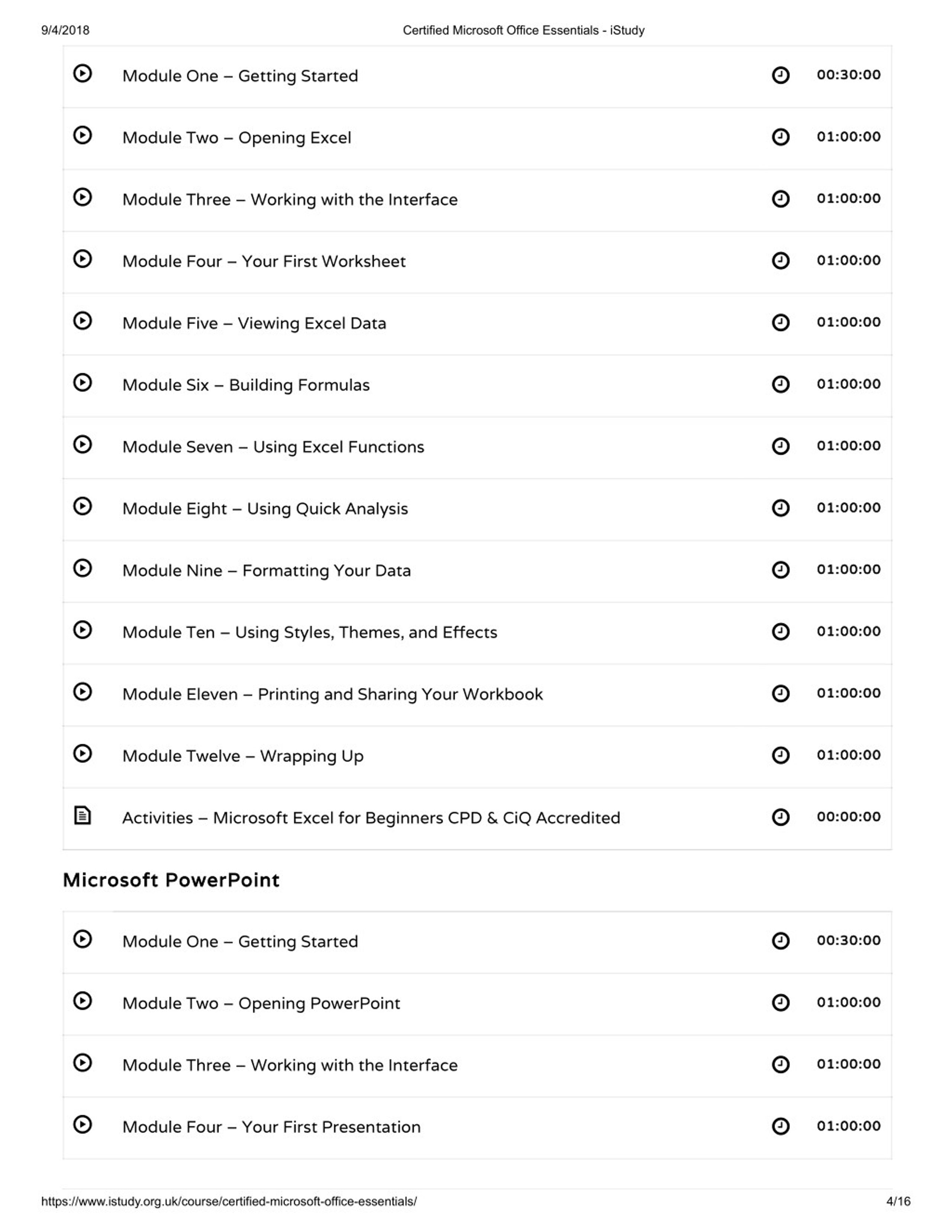Screenshot of iStudy App: Certified Microsoft Office Essentials Course (2018)

The screenshot showcases the iStudy app interface displaying a certification course titled "Certified Microsoft Office Essentials - iStudy." It specifically highlights the year 2018 on the left side. The course is structured into a series of modules:

### Modules:
1. **Module 1: Getting Started**
2. **Module 2: Opening Excel**
3. **Module 3: Working with the Interface**
4. **Module 4: Your First Worksheet**
5. **Module 5: Viewing Excel Data**
6. **Module 6: Building Formulas**
7. **Module 7: Using Excel Functions**
8. **Module 8: Using Quick Analysis**
9. **Module 9: Formatting Your Data**
10. **Module 10: Using Styles, Themes, and Effects**
11. **Module 11: Printing and Sharing Your Workbook**
12. **Module 12: Wrapping Up**

The app also features a section with additional activities:
- **Activities:**
  - Microsoft Excel for Beginners
  - CPD Accredited
  - CIQ Accredited

Each activity is accompanied by an icon of a black-and-white clock, indicating the duration of the session.

Beneath this section, the app lists modules related to Microsoft PowerPoint:
1. **Module 1: Getting Started**
2. **Module 2: Opening PowerPoint**
3. **Module 3: Working with the Interface**
4. **Module 4: Your First Presentation**

This detailed view within the iStudy app offers a comprehensive overview of the learning path for both Excel and PowerPoint basics, designed for individuals aiming to achieve proficiency in essential Microsoft Office tools.